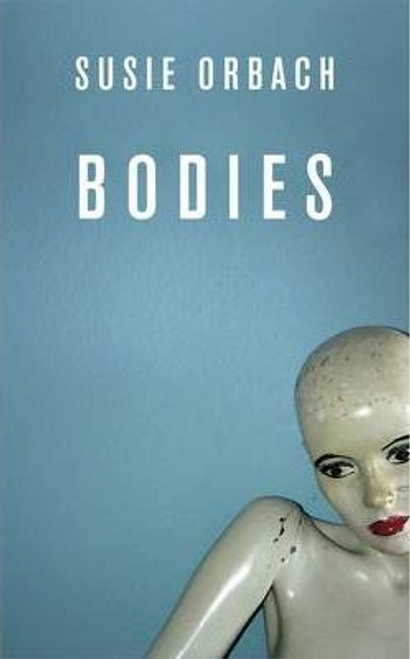The image is a vertical book cover with a cool, somewhat faded blue background. At the top of the cover, in a narrow white font, it reads "SUSIE ORBACH," the author's name, in all capital letters. Just below, in a larger, spaced-out white font, also in all capitals, is the book's title, "BODIES." Dominating the lower right corner of the cover is an unclothed female mannequin with a grayish-tan, shiny complexion. The mannequin's surface appears worn, featuring visible cracks on the shoulder and head, along with several nicks and scrapes. It has striking facial features, including red lipstick, black eyeliner, thick eye makeup, and dark eyebrows, but lacks hair. The background and design remain minimalistic, drawing attention to the mannequin’s compelling, imperfect form.